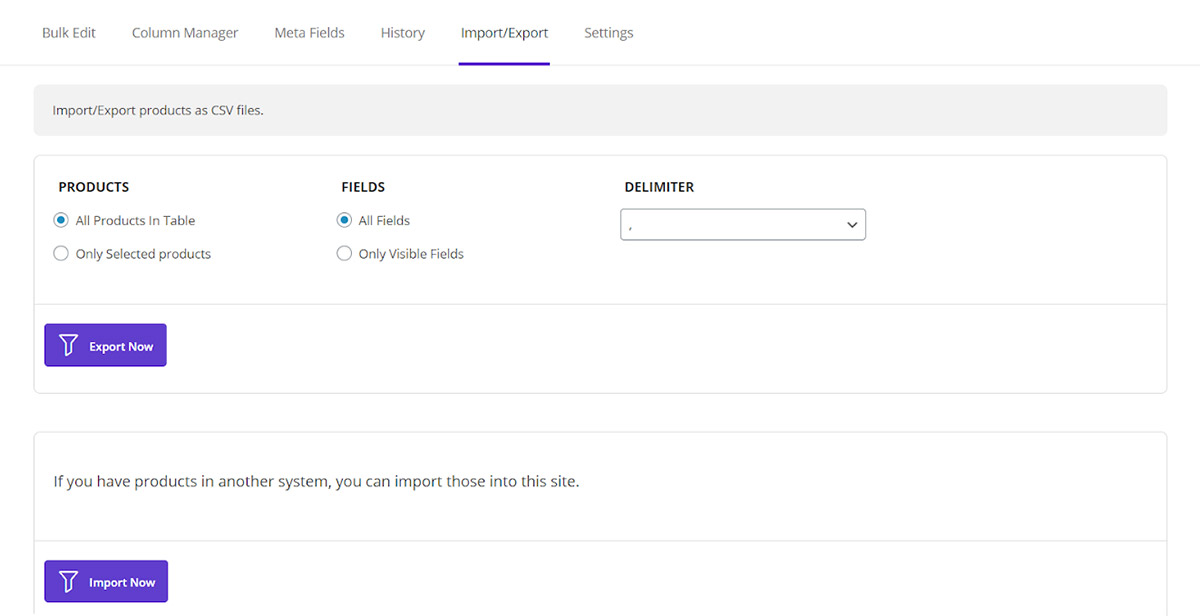This webpage features various options and filters accompanied by a predominantly white background, accented with purple buttons and grey sections. At the top, there are multiple fields, each designated for different functions: "Bulk Edit," "Column Manager," "Meta Fields," "History," "Import/Export," and "Settings." The "Import/Export" field is highlighted with a purple underline to indicate it is currently selected.

Below these fields, a grey bar displays the text "Import Export Products as CSV Files." Beneath this bar, there are three main sections: Products, Fields, and Delimiter. 

1. **Products Section:**  
   - "All Products in Table" (selected with a blue circle) 
   - "Only Selected Products"

2. **Fields Section:**  
   - "All Fields" 
   - "Only Visible Fields"

3. **Delimiter Section:**  
   - A blank input box

Additionally, a noticeable purple "Export Now" button allows users to export the selected data immediately.

Further down the page, a dedicated import section invites users to import products from other systems into this site. This section includes an "Import Now" button with a purple background for easy access.

Overall, the page is designed to facilitate the efficient management and transfer of product data through a user-friendly interface composed of well-defined sections and intuitive options.